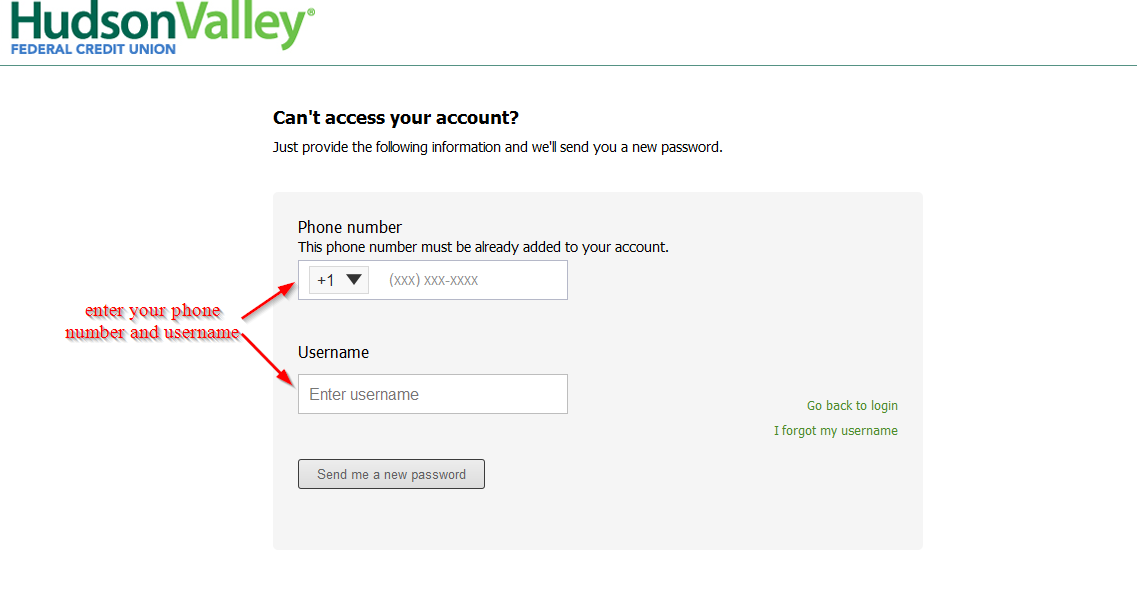In this image, we see a screenshot from the Hudson Valley Federal Credit Union website. At the top left corner, the words 'Hudson' and 'Valley' are displayed, with 'Hudson' in dark green and 'Valley' in a lighter green color. Just below this, 'Federal Credit Union' appears in blue text.

Centrally located on the page is a message that reads, "Can't access your account? Just provide the following information and we will send you a new password." Below this instruction, the form requests a phone number, stating that "This phone number must already be added to your account." There is a white rectangle field to input the country code followed by the rest of the phone number in the format (XXX) XXX-XXXX.

Underneath the phone number field, there is a field for a username with a white rectangle placeholder that says "Enter username." Beneath these fields is a gray button labeled "Send me a new password."

On the right side of this information box, there is green text that provides additional options: "Go back to login" and "I forgot my username."

Additionally, someone has added instructional text near these fields: "Enter your phone number" next to the phone number field and "Enter your username" next to the username field. Red arrows point to these corresponding input boxes for clarity.